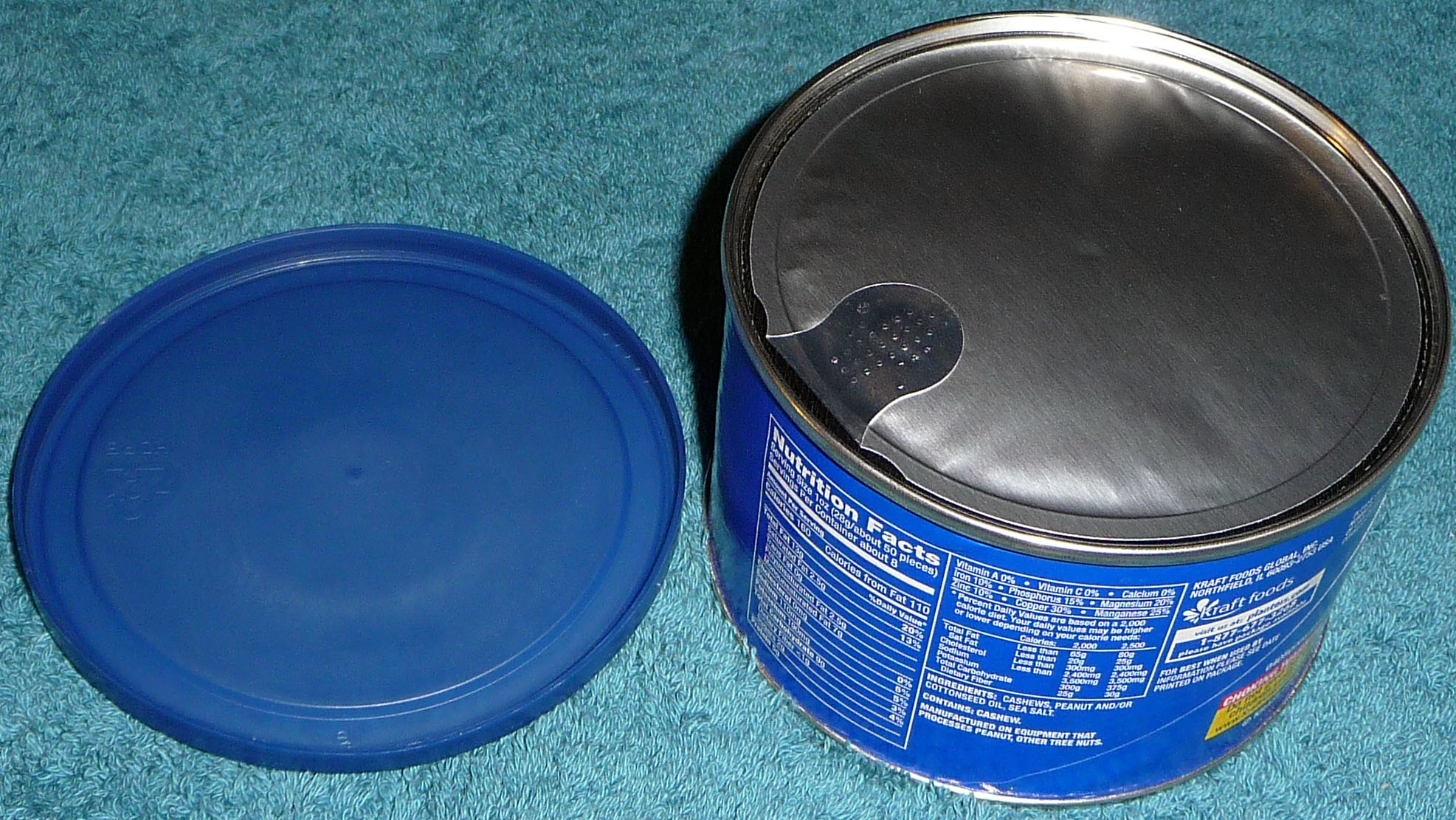A bright blue can of coffee is prominently displayed on a plush, blue shag rug. The can's plastic cover, removed and placed to the left, reveals the bottom of the container. The coffee is still sealed with a shiny silver Ziploc cover, complete with a pull tab for easy opening. The canister, shown from the back, features a white nutritional facts table. A yellow rectangle near the base adds a splash of contrasting color to the scene. Dominant hues in the photograph include various shades of blue, shimmering silver, and crisp white, creating a visually striking composition.